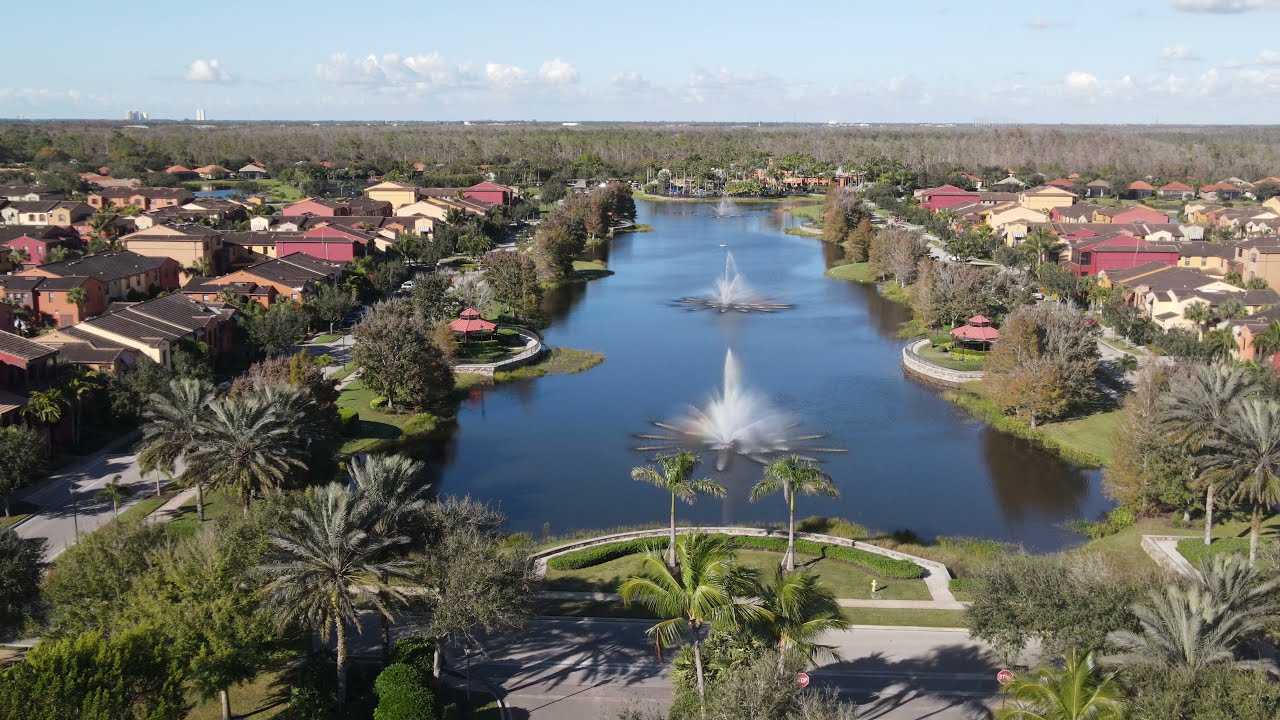This detailed aerial view captures a picturesque community nestled around a serene lake. The lake, situated centrally, features three distinct water fountains that shoot white water into the air, creating a dynamic focal point. The banks of the lake are framed by manicured lawns, green trees, and various bushes, enhancing the meticulously maintained landscape. 

Palm trees dominate the foreground, adding a tropical touch, while a gray sidewalk winds through, lined with more greenery, underlining the neighborhood's tranquility. Flanking the lake are rows of houses in hues of red, white, yellow, and tan, with roofs mostly in dark brown or black. These houses, consistent in their neat appearance, are interspersed with additional greenery, adding layers of color and texture.

The backdrop reveals a horizon of densely wooded areas, featuring tall brown and gray trees, which blend into the light blue sky dotted with wispy white clouds. This idyllic scene embodies the essence of a peaceful, well-kept suburban enclave under a clear, daytime sky.